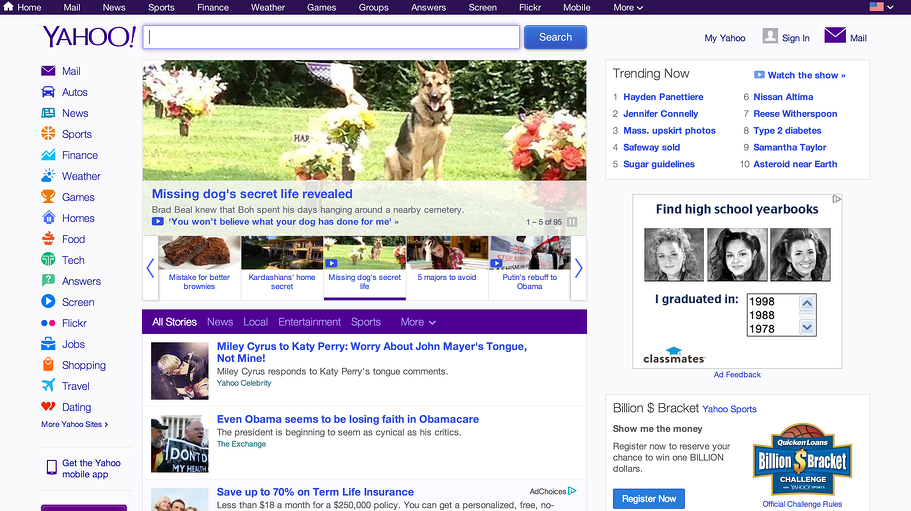A detailed screen capture from the Yahoo homepage reveals a gray background interspersed with black text and vibrant purple accents characteristic of Yahoo’s theme. The top of the page features a black navigation bar with white text offering links to "Home," "Mail," "News," "Sports," "Finance," "Weather," "Games," "Groups," "Answers," "Screen," "Flickr," "Mobile," and a "More" dropdown menu. In the top right corner, an American flag icon with a dropdown menu suggests options for changing the region or language settings.

On the upper left, the iconic Yahoo logo is prominently displayed alongside icons that mirror the top menu's categories. Centrally positioned is a search bar designed for quick information retrieval.

The main content region hosts a series of news articles. One headline reads "Missing Dog's Secret Life Revealed" and is accompanied by an image of a German Shepherd seated in a cemetery. Additional articles populate the page’s central column, offering various news stories.

The right column highlights trending topics and features an advertisement for Classmates.com, promoting high school yearbook searches. This ad includes images of women possibly from the 1980s, paired with statements like "I graduated in 1998," "I graduated in 1988," and "I graduated in 1978." Another ad on the page promotes "Billion Brackets."